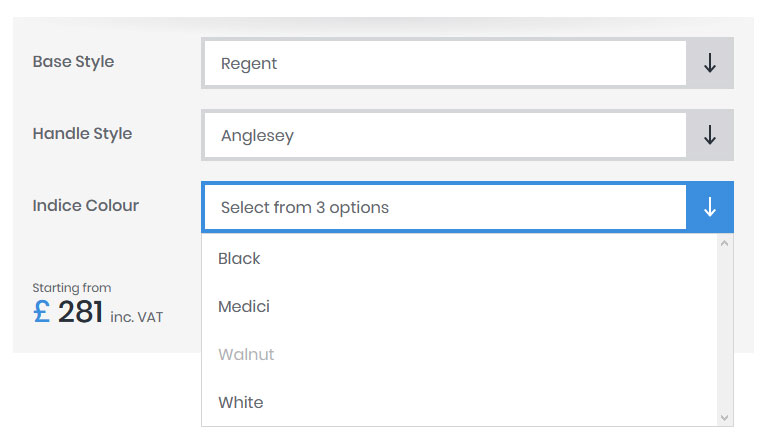Screenshot of a Customization Panel:

The image displays a cropped section of a customization panel set against a gray background, highlighting three customization options. In the top left corner, "Base Style" is labeled in dark gray letters. To the right, a large drop-down box shows "Regent" as the selected option. Below this, "Handle Style" is labeled on the left with another large drop-down box to the right, showing "Angel Sea" as the selected option.

Further down, the label "Indus Color" appears on the left, accompanied by a drop-down box on the right that is currently highlighted in blue, indicating that it is active. The box invites the user to "Select from three options" and displays a drop-down menu with four options. However, the option for "Walnut" is grayed out and marked as sold out. The available options for selection are "Black," "Medicine," and "White."

At the bottom left corner of the panel, text indicates that prices start from $281, including VAT.